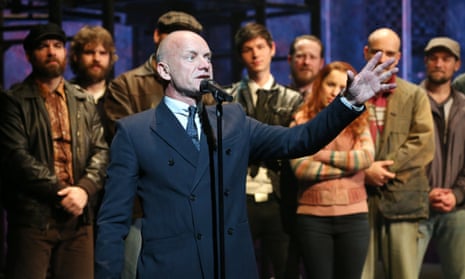In this detailed photograph, we see a mostly bald man standing at the forefront on what appears to be a stage, addressing an audience through a black microphone on a stand. He is impeccably dressed in a blue suit with a blue tie and a white shirt, and his left hand is extended upwards, depicting an animated moment of speech. The man in the picture bears a striking resemblance to the singer Sting. Behind him, an assembly of predominantly younger individuals, likely college students, are visible. Among them, only one woman stands out; she has ginger hair and is wearing a pink sweater with striped sleeves and black trousers. The rest of the group is composed entirely of men, dressed variably in casual, somewhat drab clothing ranging from black hats, brown leather jackets, plaid flat caps, to worn brown coats. They all stand attentively, eyes fixed on the speaker, giving off an air of respect and concentration, possibly indicating that the man is either making an important announcement, introducing a play, or concluding a significant event. The background is a shade of blue, reinforcing the formal and staged setting of this engaging scene.